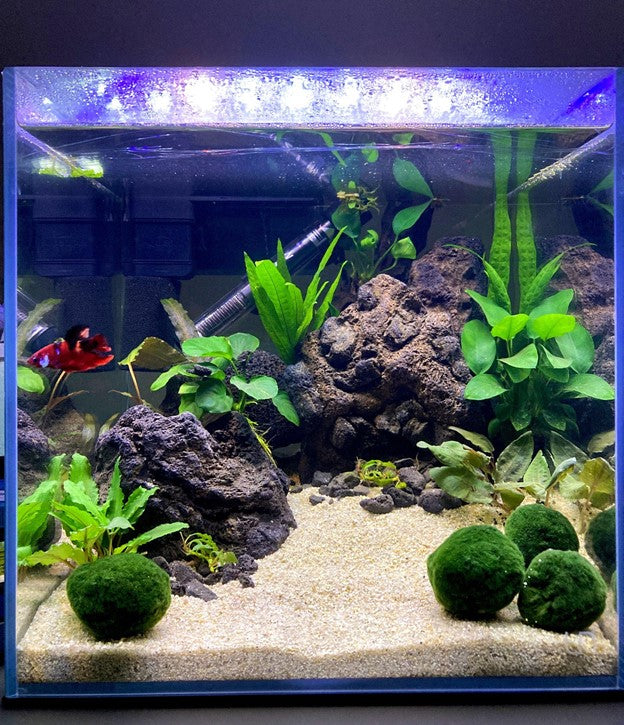This detailed photograph of an aquarium reveals a meticulously arranged aquatic scene set indoors. The aquarium borders are outlined in blue-tinted acrylic with noticeable condensation above the waterline. It sits on a dark gray platform and is illuminated by artificial lighting that casts a serene blue glow across its contents. Inside, a landscape of beige, fine-grained sand forms the substrate, scattered with large, brown rock formations. Among these formations, green aquatic plants with lush leaves provide a vivid pop of color and natural habitat. A prominent feature at the back of the tank is a long, pipe-like water filter.

Dominating the left side of the scene is a small, vibrant red betta fish, its tail pointed and elegantly flowing as it swims toward the left side of the image. Floating near the surface of the water is a cluster of green algae or plant matter. The overall setting of the aquarium is immersive, offering a tranquil underwater vista enclosed within a rectangular frame that measures approximately six inches high and four inches wide. Despite the presence of various objects and plant life, the solitary red betta fish remains the focal point of this peaceful aquatic environment.